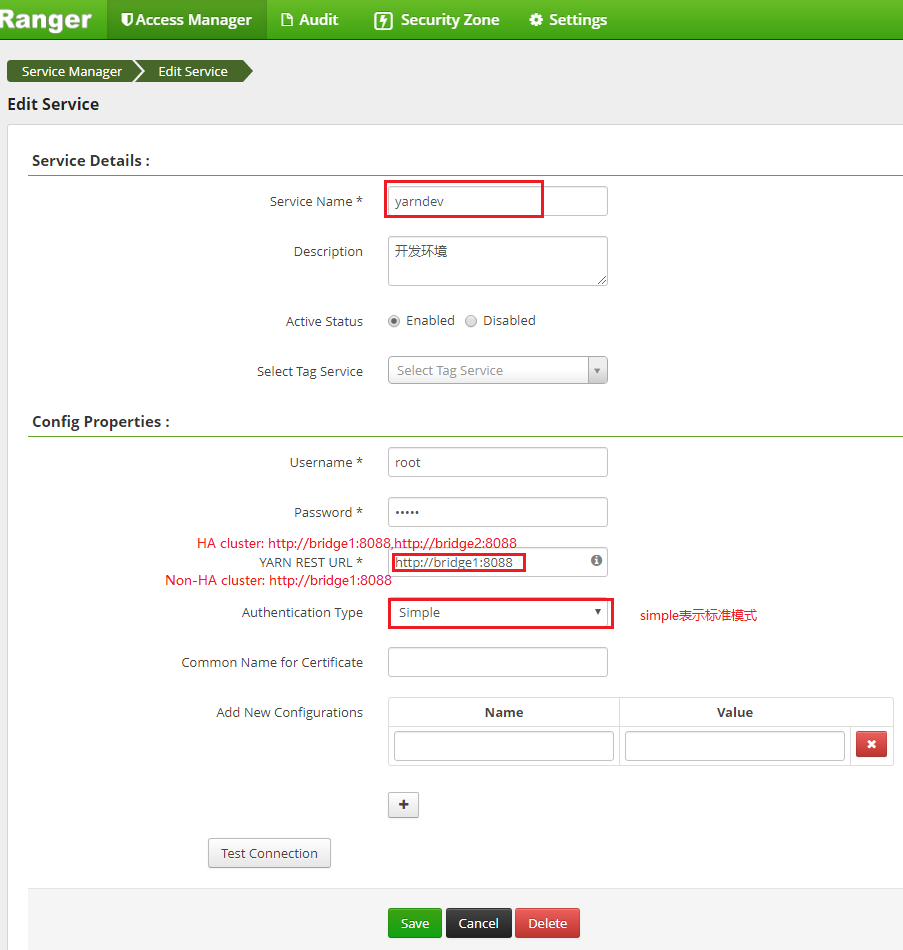This image depicts the interface of a website named "Ranger." The top section features a blue banner with several options: Access Manager, Audit, Security Zone, and Settings. Below this, the layout displays sections for Service Manager, Edit Service, and Edit Service Details. Users can input their service name and provide a description of the issue in designated fields.

A status indicator shows the service as "Enabled," with an option to toggle between active and disabled states. Additionally, a "Select Tag Service" option is available. Configuration properties include fields for a username, displayed as 'root,' and a password field that is masked. A Yarn Rest URL is specified as "http://bridge18088" under a labeled configuration panel.

The interface supports simple authentication, visually marked within a red square, and leaves the "Common Name for Certificate" field blank. Notably, the interface displays text in both Chinese and English.

At the bottom of the configuration panel, there's an "Add New Configurations" option with fields to input 'Name' and 'Value,' alongside a plus button to add entries. There's also a "Test Your Connection" button for verifying configurations. Finally, the bottom section of the page offers options to Save, Cancel, or Delete the entered configurations.